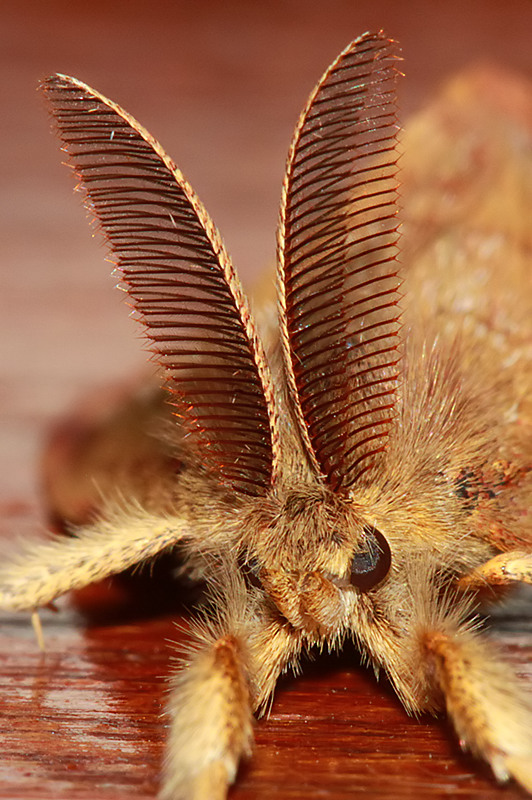This close-up photograph captures the intricate details of a fuzzy, tawny brown moth perched on a wooden surface. The moth's bulbous eyes dominate its head, flanked by two large, comb-like antennae that fan out horizontally and curve gently, resembling the structure of a feather with dozens of fine, dark brown strands. These impressive antennae meet near the center of the insect's head, giving an appearance similar to parasailing sails or satellite dishes. The moth's body is enveloped in light and dark brown fur, adding to its hairy texture. Its wings, held upright, are long ovals featuring horizontal lines that give a see-through effect, showing glimpses of its body beneath. The moth's legs are visible, with two outstretched in front and additional legs extending to the sides. The background is artistically blurred, placing the focus squarely on the moth's detailed features.